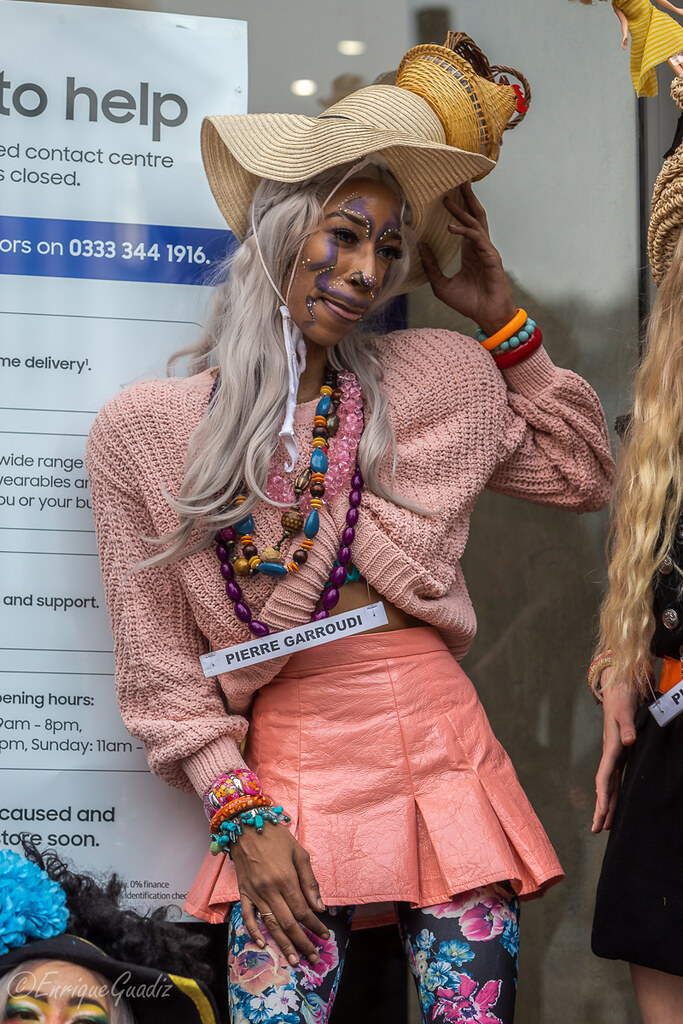In this vibrant outdoor daytime portrait, a tall, slender woman of African descent stands in front of a poster with visible text including “to help” and “contact center closed.” The woman, who is posing in the center from mid-thigh up, has her face intricately painted with a striking combination of violet, white, purple, and gold. Violet and white paint decorates her eyes, cheeks, and upper lip, while her nose is highlighted with gold and black. Her hair, dyed in a purplish-silver hue, is styled with a braid around the top of her head, cascading down past her shoulders.

She sports a unique hat ensemble: a large, floppy straw hat topped with a smaller straw hat adorned with a wicker basket from which a wicker chicken emerges. Her attire includes a peach-colored sweater that emphasizes her midriff and a pink leather mini skirt. Adding to her eclectic style, she wears a plethora of large bead necklaces in colors such as purple, blue, yellow, and orange, along with similarly colored bracelets on both wrists. She stands against a background featuring parts of a banner with phrases like "to help," a contact number, and other partially visible text related to an awareness event.

On the left side of the image, a person of Caucasian descent is partially visible, characterized by a black hat with black feathers and a blue plume. Their face is adorned with a watermark reading "copyright Enrique G-U-A-D-I-Z." Additionally, another individual with long blonde hair is partially shown on the right, wearing a black skirt and a hat. This highly detailed and whimsical composition encapsulates an eclectic and colorful scene brimming with creative expression and unique fashion elements.